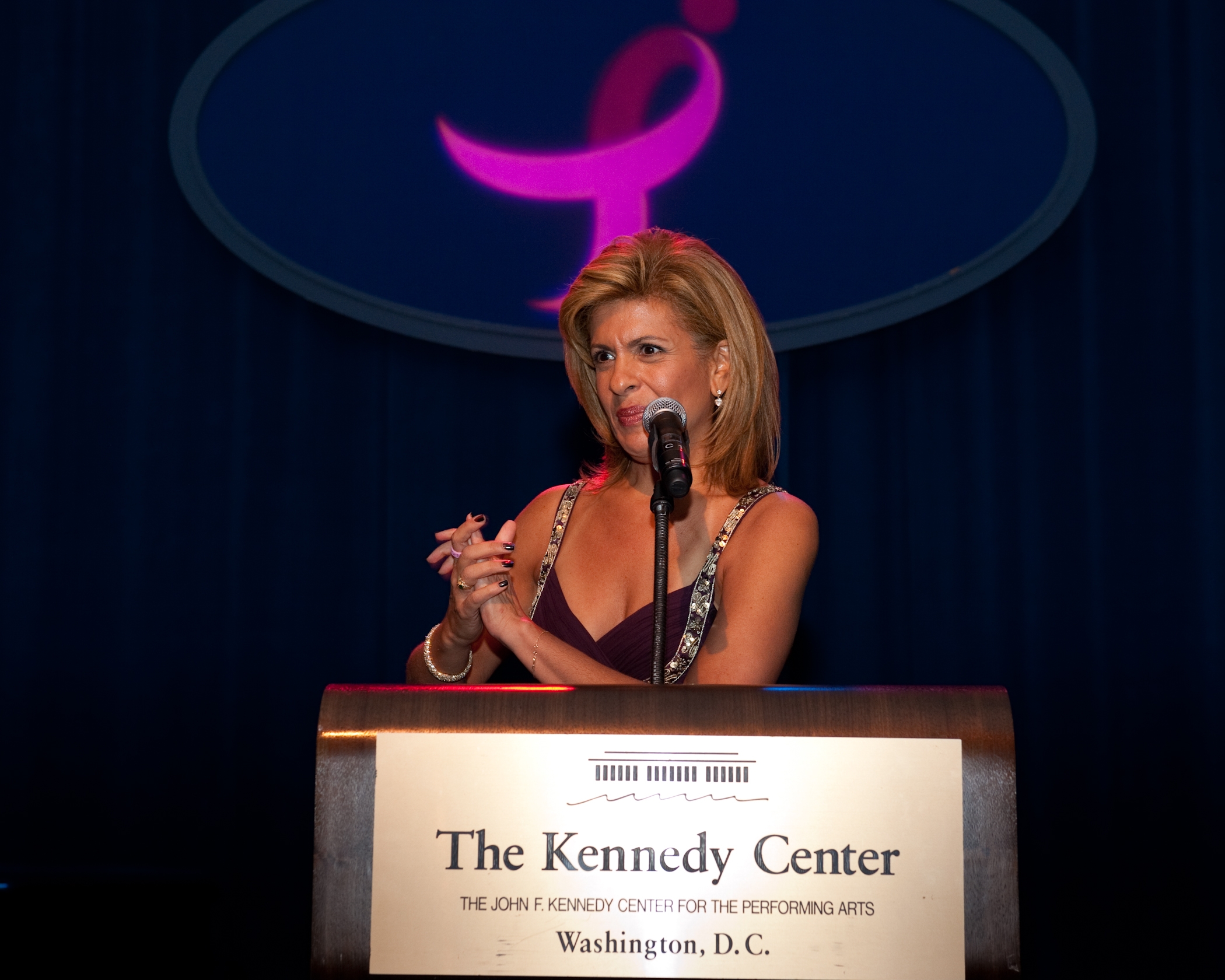In this detailed color photograph, a woman stands at a dark wood podium with a bronze-colored plaque labeled "The Kennedy Center, The John F. Kennedy Center for the Performing Arts, Washington, D.C." prominently displayed in black lettering. A black microphone with a silver round end is attached to a black microphone stand and is pointed towards her face. The woman, whose blonde hair is styled into a shoulder-length bob parted in the middle, is dressed in a thin-strapped, v-neck red dress with sparkling shoulder accents. She wears a gold bracelet adorned with multiple jewels and has her nails painted black. Her hands are clasped together in front of her, revealing multiple rings. Notably, she also wears dangling earrings that catch the light. Behind her is a blue curtain wall adorned with a large blue oval symbol, within which there is a cursive pink letter 'L'. The background and elements highlight her poised stance as she looks out into the audience, slightly towards her left, with a composed expression. The overall ambiance is enhanced by lights that create a subtle pink glare on her shoulder.